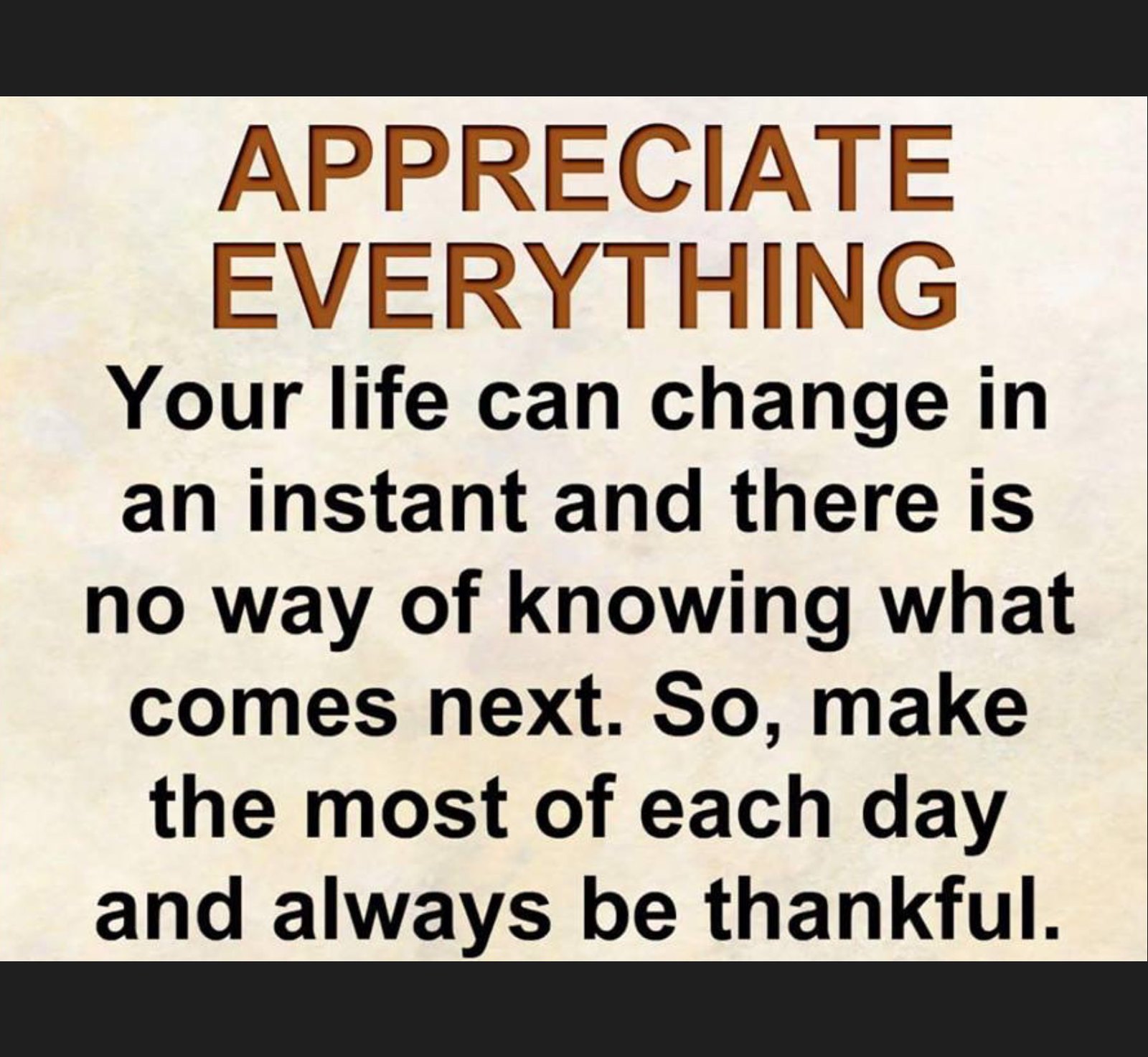The image is a motivational poster typically seen on platforms like Facebook. It features a tan and textured light pink background with a creamy white hue. The design is framed with black letterbox borders at the top and bottom. The central message in big, bold orange letters says, "Appreciate Everything." Below this, in black lettering, the poster continues with, "Your life can change in an instant and there is no way of knowing what comes next, so make the most of each day and always be thankful." The text is presented with normal capitalization, emphasizing the importance of gratitude and mindfulness.